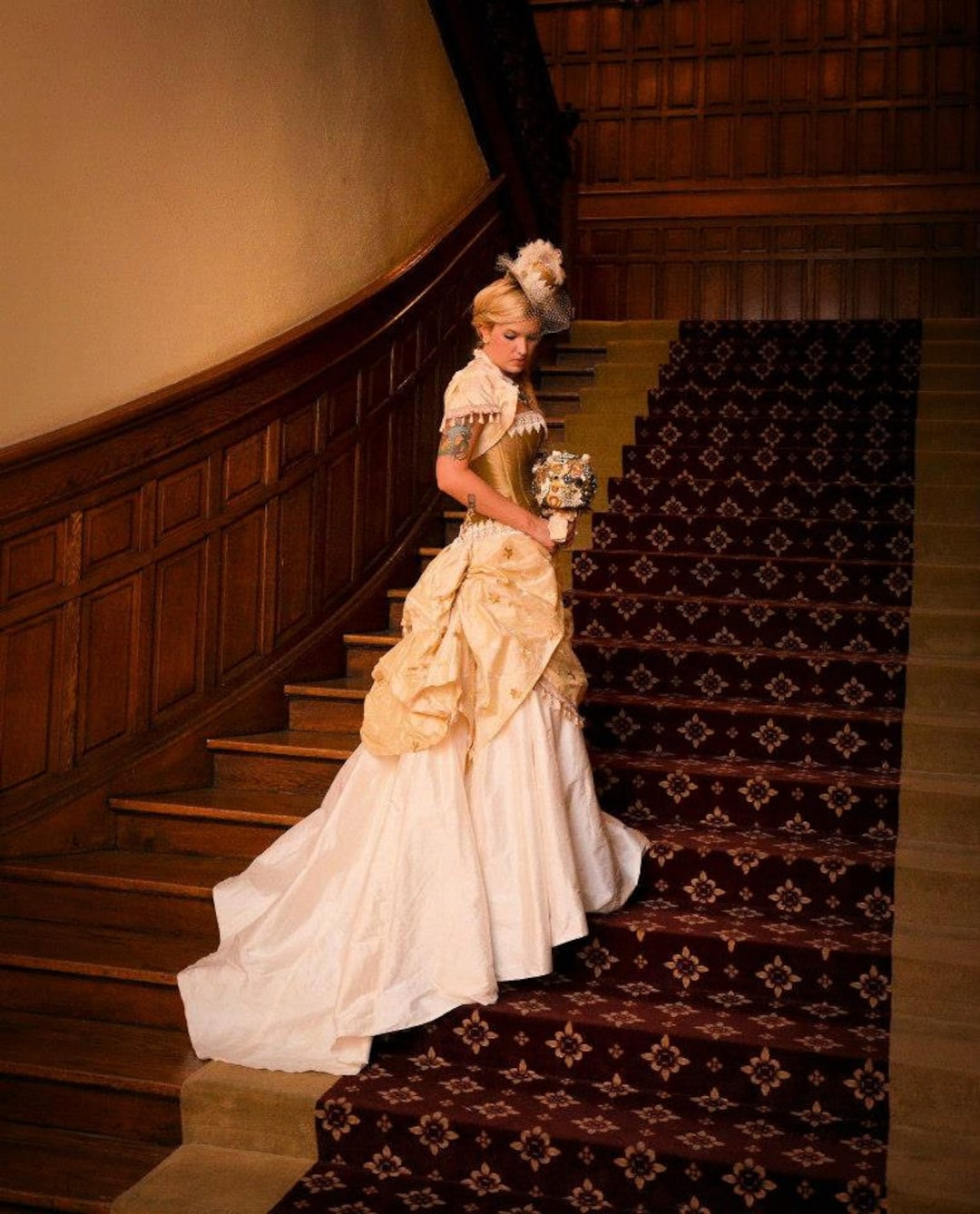The image depicts a young woman with blonde hair styled in a bun, dressed in an elegant off-white, mid-19th century style gown with a shiny gold bodice. The dress is adorned with an ivory-colored overlay and features short sleeves. She holds a bouquet of flowers and wears a hat decorated with flowers. The scene takes place on a grand, wooden staircase that is at least six to eight feet wide. The staircase is covered by a patterned carpet runner in dark red and black, not extending to the outer edges, revealing the wooden steps. The staircase is flanked on the left by a wall with wooden paneling at the bottom and white plaster above. The woman is ascending the stairs, looking down and to her right, where more light illuminates the scene compared to the right side. The top of the staircase and part of the landing are visible in the background.